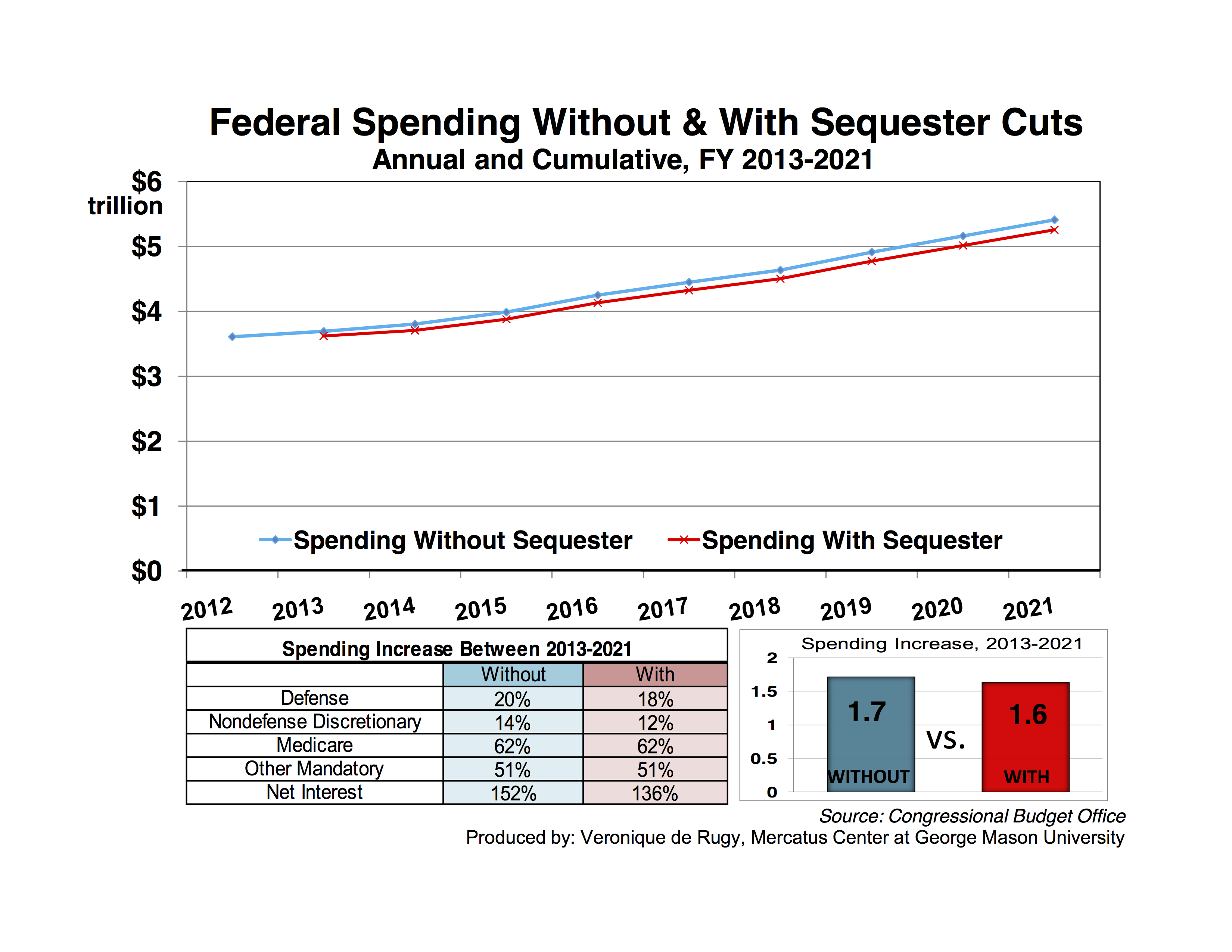The image displays a bar graph illustrating federal spending from fiscal year (FY) 2013 to 2021, highlighting the impact of sequester cuts. The vertical axis ranges from $0 to $6 trillion, while the horizontal axis spans the years from 2012 to 2021.

The top portion of the graph features blue bars representing spending without sequester cuts and red bars for spending with sequester cuts. Both sets of bars run almost parallel to each other, indicating minimal differences between the two scenarios. The spending per year varies from approximately $350 billion to about $5.5 trillion over the examined period.

Additional text on the image details specific spending categories and their respective increases during this timeframe. For instance, defense spending is projected to increase by 20% without sequester cuts but only by 18% with them. Non-defense discretionary spending would see a 14% increase without the sequester and a 12% increase with it. Medicare is expected to rise by 62% in both scenarios, while other mandatory spending shows a 51% increase regardless of sequester cuts. Net interest spending is projected to grow by 152% without sequester, compared to 136% with it.

In summary, the graph indicates that the total spending increase from 2013 to 2021 is 1.7 times without sequester cuts and 1.6 times with them, suggesting that sequester cuts have a relatively negligible impact on the overall spending trajectory.